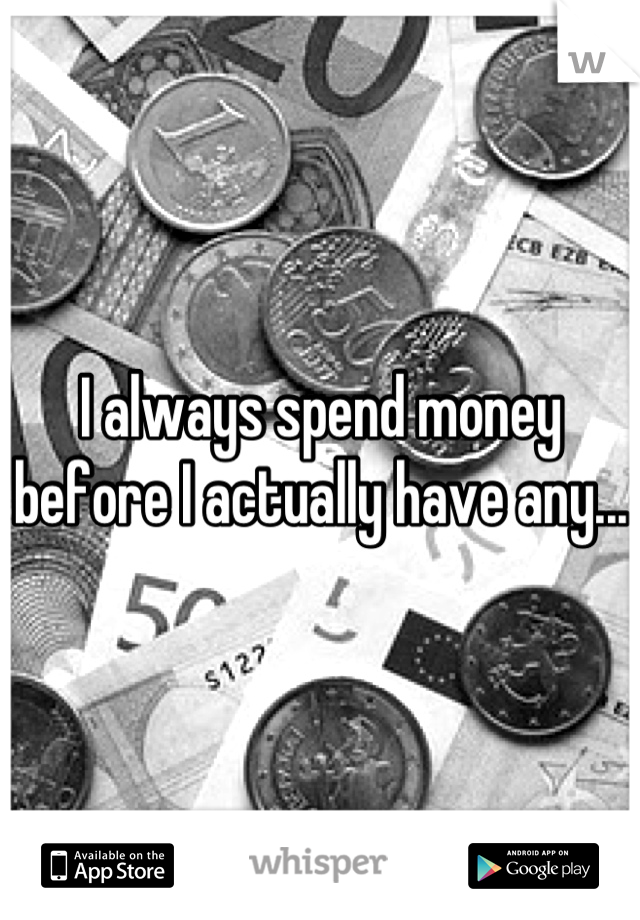The grayscale portrait-oriented image features a scattered array of various types of currency, primarily non-US coins and paper bills. Several coins display the denominations 1, 50, and 2, while the overlapping paper money features the numbers 2, 50, 10, and 20 alongside visible serial numbers. Centered prominently in the image is a meme with white text outlined in black that reads, "I always spend money before I actually have any..." At the bottom, three icons are lined up: on the left is the "Available on the App Store" icon, in the middle is the gray text "whisper," and on the right is the Google Android app icon. The black-and-white photo is realistic with a touch of typographic elements designed for social media sharing.